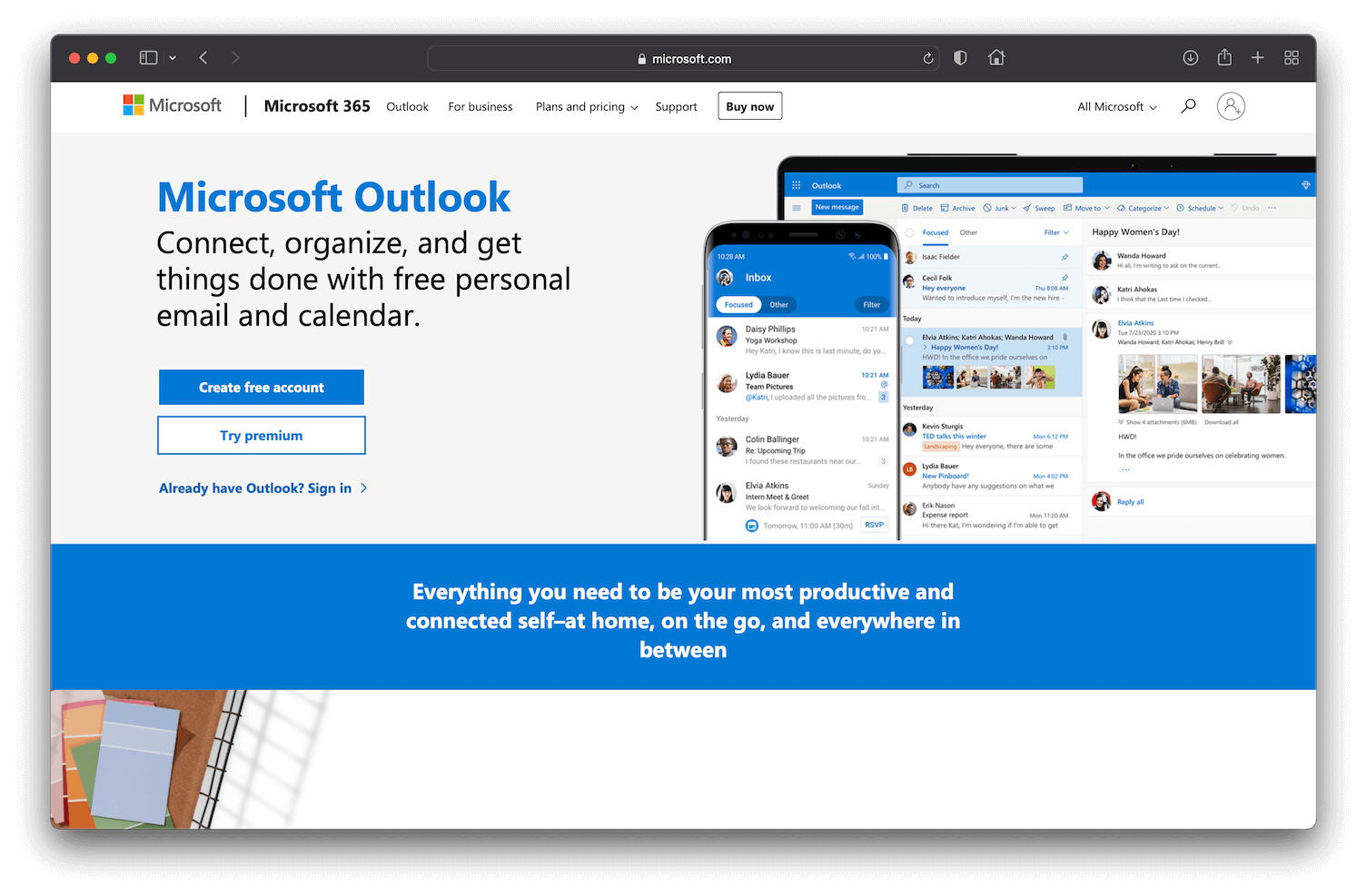The image depicts the Microsoft Outlook web interface, seemingly set up for a free account. The top navigation bar includes a variety of features: a search bar labeled "Microsoft.com," a refresh button, a partially colored badge, a home button, a download icon, a "send plus" option, and a grid of four squares. A back button is positioned on the far left.

In the upper left corner, the presence of the red, yellow, and green buttons indicates that the interface is displayed on an Apple device. Below these buttons is the Microsoft emblem featuring red, green, orange, and blue squares.

Highlighted on the interface is a bolded monthly plan cost of $3.65, aimed at users considering a subscription plan. Adjacent to this is a section titled "Outlook for Business Plans," accompanied by a dropdown for plan and pricing options, as well as a support link. A "Buy Now" button is also visible.

To the far right, there's a dropdown menu labeled "All Microsoft," a search icon, and a username placeholder indicating that no one is currently logged in. 

Below the primary navigation bar, there is a prominent advertisement banner for Microsoft Outlook. The Outlook name is displayed in large blue font. The tagline underneath reads, "Connect, organize, and get things done with free personal email and calendar." 

Two distinct action buttons are positioned below this tagline: a blue button with white text that says "Create Free Account" and a white button with blue text that says "Try Premium." There is also a smaller link reading "Already have Outlook? Sign in."

To the right of this section, there are visual depictions of the Outlook interface on both a laptop and a smartphone, illustrating how users can manage emails and previews across devices. 

At the very bottom, a wide blue banner emphasizes the service's benefits: "Everything you need to be your most productive and connected self at home, on the go, and everywhere in between."